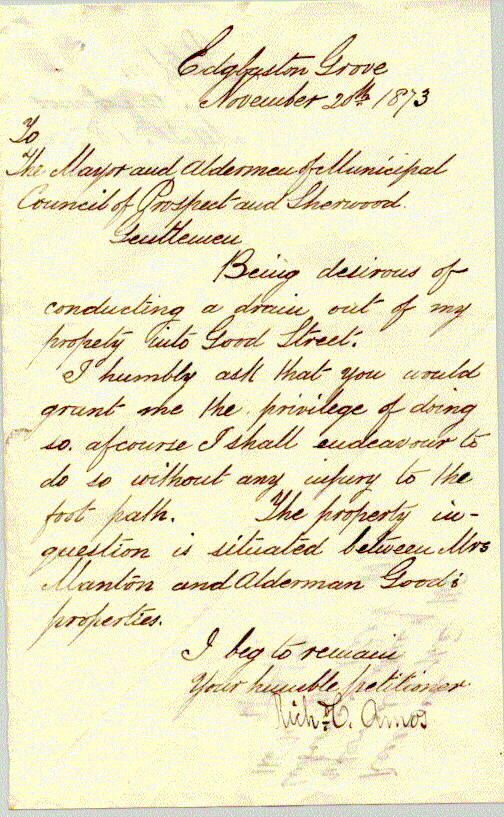This image depicts an old, handwritten letter dated November 20th, 1873, addressed to the Mayor and Aldermen of the Municipal Council of Prospect and Sherwood. The letter is written in cursive on a worn, yellowish parchment-like paper with brownish-black ink. The document is standard paper size and placed on a grey surface. At the top, the address "Edgerton Grove" is visible. Despite the text being difficult to decipher, the body of the letter appears to be a formal request for permission to conduct a drain from the author's property onto Good Street. The author emphasizes their intent to avoid causing any damage to the pathway. Furthermore, the property in question is described as being situated between "Mrs. Mansion" and "Alderman Good's properties." The letter concludes with a humble petition, signed by an individual whose name seems to be "Rich Amos."